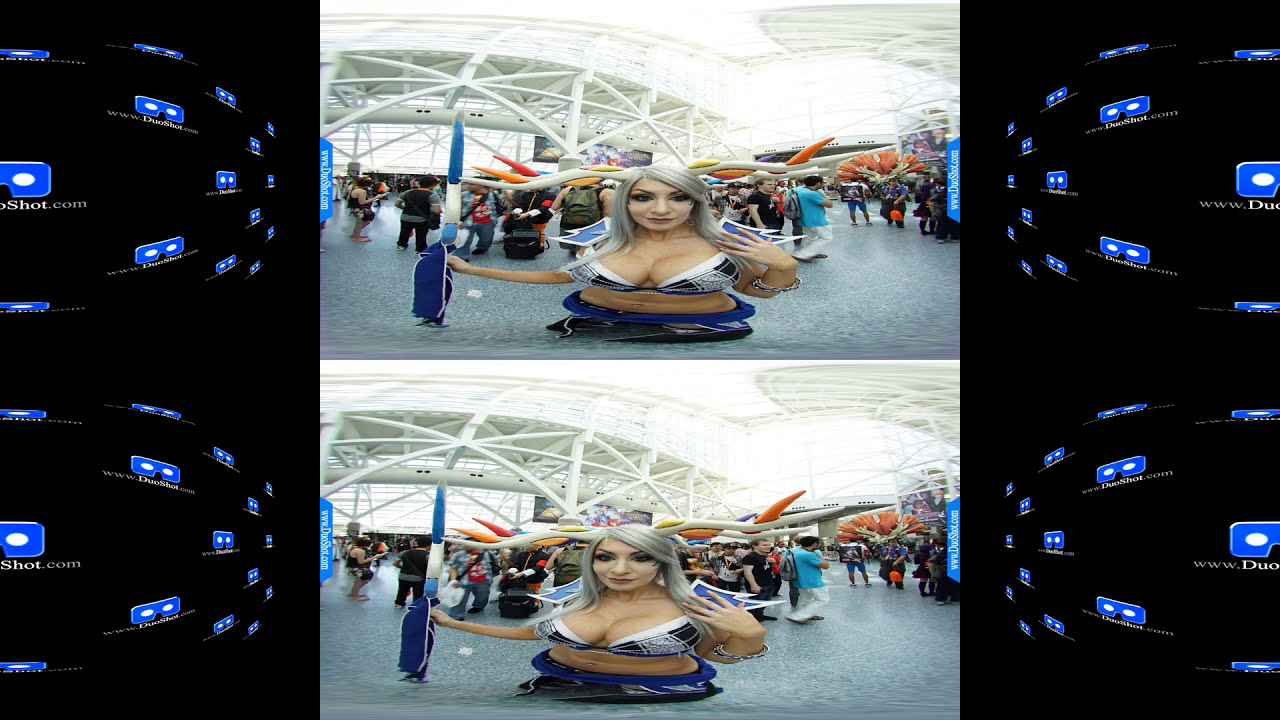This screenshot captures two vertically stacked photographs featuring a cosplay model at a large convention hall, bustling with people. The images, almost identical, are bordered by a black background featuring a logo that resembles a pair of black 3D glasses with white lenses and the URL www.duoshot.com. The model, likely in her late 20s or early 30s, has strikingly arranged silver hair resembling antlers or branches, with tips colored red, yellow, and orange. She is dressed in a blue bikini top and blue bottoms, exposing her midriff. In one hand, she holds a blue, white, and teal scepter, adding to her elaborate costume. The overall scene suggests a vibrant and busy cosplay fair, further enriched by her detailed and imaginative attire.